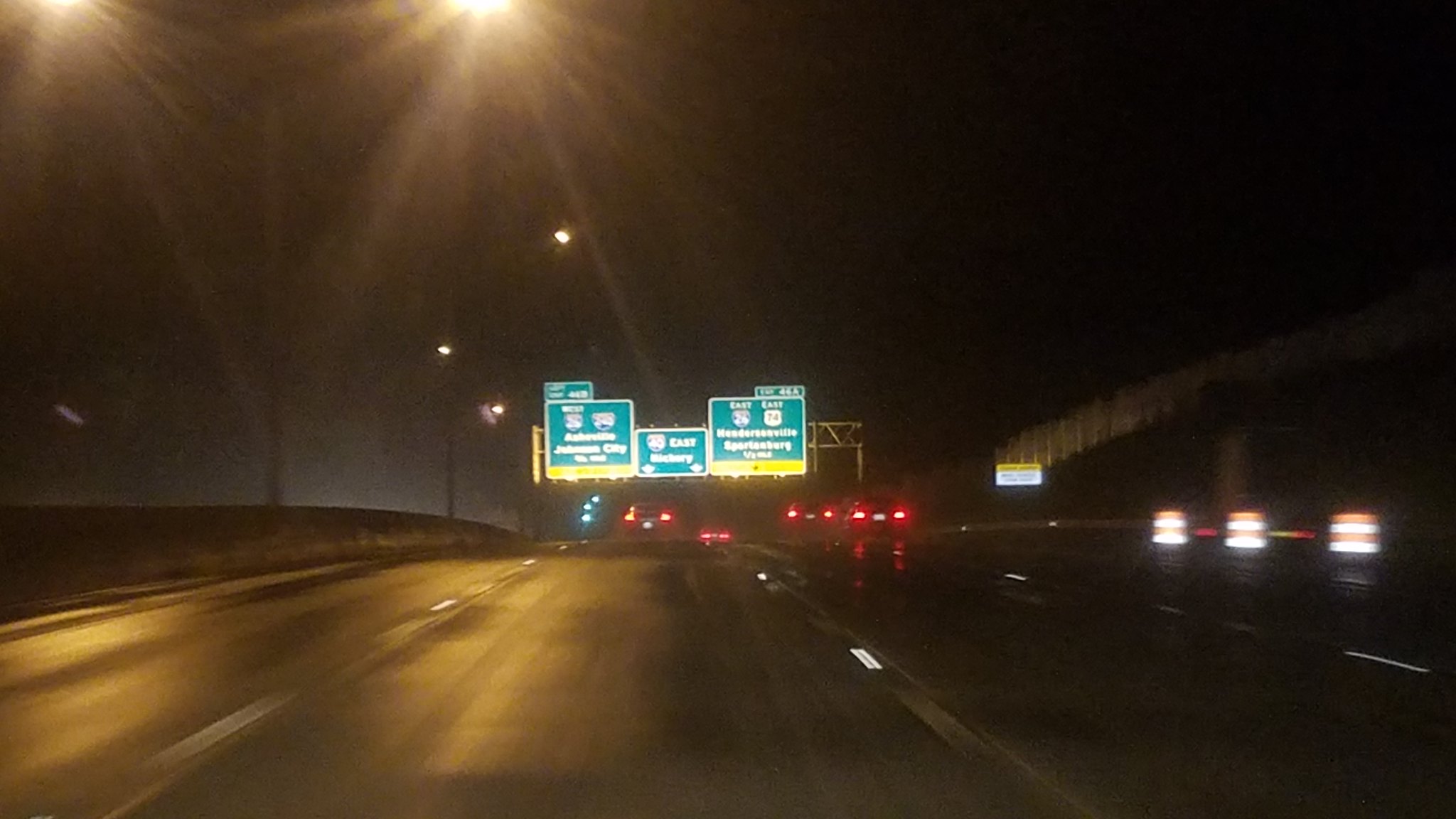A nighttime photograph captured from the interior of a car through the windshield, showcasing a dimly lit road. In the distance, three green highway signs are visible, stacked side by side, indicating upcoming exits. Although partially obscured, the signs display city names such as "Johnson City" and directions like "East." The road features white lane markers, guiding the way. Ahead, four cars are visible: one in the same lane as the viewer’s vehicle and three in the adjacent lane. The image conveys the stillness and focused visibility essential for nighttime driving on a highway.